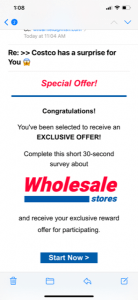A person is viewing a suspicious message on their smartphone, purportedly from Costco. The phone's screen displays the time, battery life, and good connection status. The time shows 1:08, and a gray bar indicates an active item in the cart. On the left side, there's a blue circle with an arrow pointing left. Below this, an unreadable blue text is present. At 11:04 a.m., in bold black letters, the message reads "RE: Costco has a surprise for you," accompanied by a surprise emoji. The notification, highlighted by a red "Special Order Offer" bar, invites the recipient to complete a 30-second survey about wholesale stores, promising an exclusive reward. The word "Congratulations!" appears in black with an exclamation point. The message ends with a blue "Start Now" box. Key identifiers such as legitimate branding from Costco are missing, suggesting the message is a scam. The text "wholesale stores" is displayed in red and blue, further indicating the lack of authenticity.